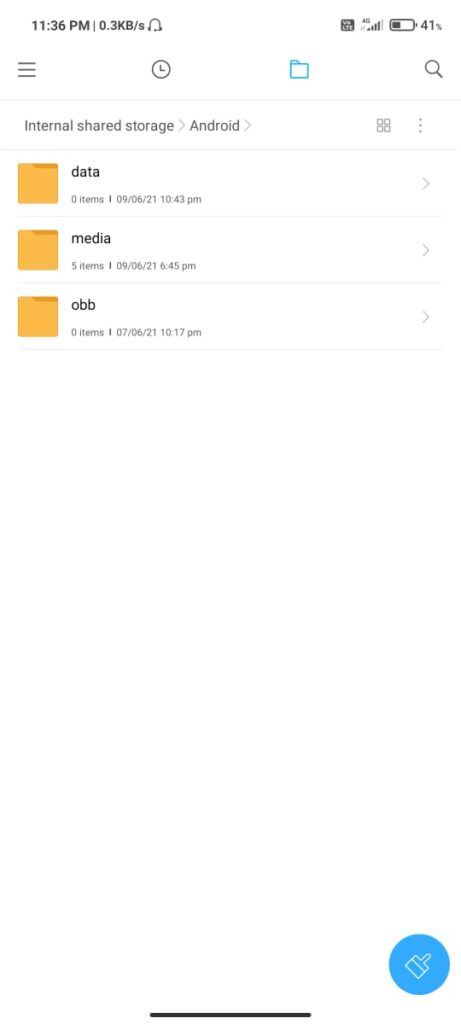The image depicts a mobile app interface, specifically a file manager on an Android phone. At the top of the screen, there's a navigation path indicating that the current directory is within the "Internal Shared Storage" and the "Android" subfolder. Within this "Android" folder, three additional folders are visible: "Data," "Media," and "obb." Both "Data" and "obb" folders appear to be empty, while the "Media" folder contains five items. The details on the screen show that the last modification or addition to the "Media" folder occurred on September 6th, 2021, at 6:45 PM. The interface features a clean, white background, with not much extraneous detail. In the status bar at the top of the screen, various indicators are visible: the battery is at 41%, the device is connected via 4G LTE, the current time is 11:36 PM, and there's an icon suggesting that headphones (either wired or Bluetooth) are connected.